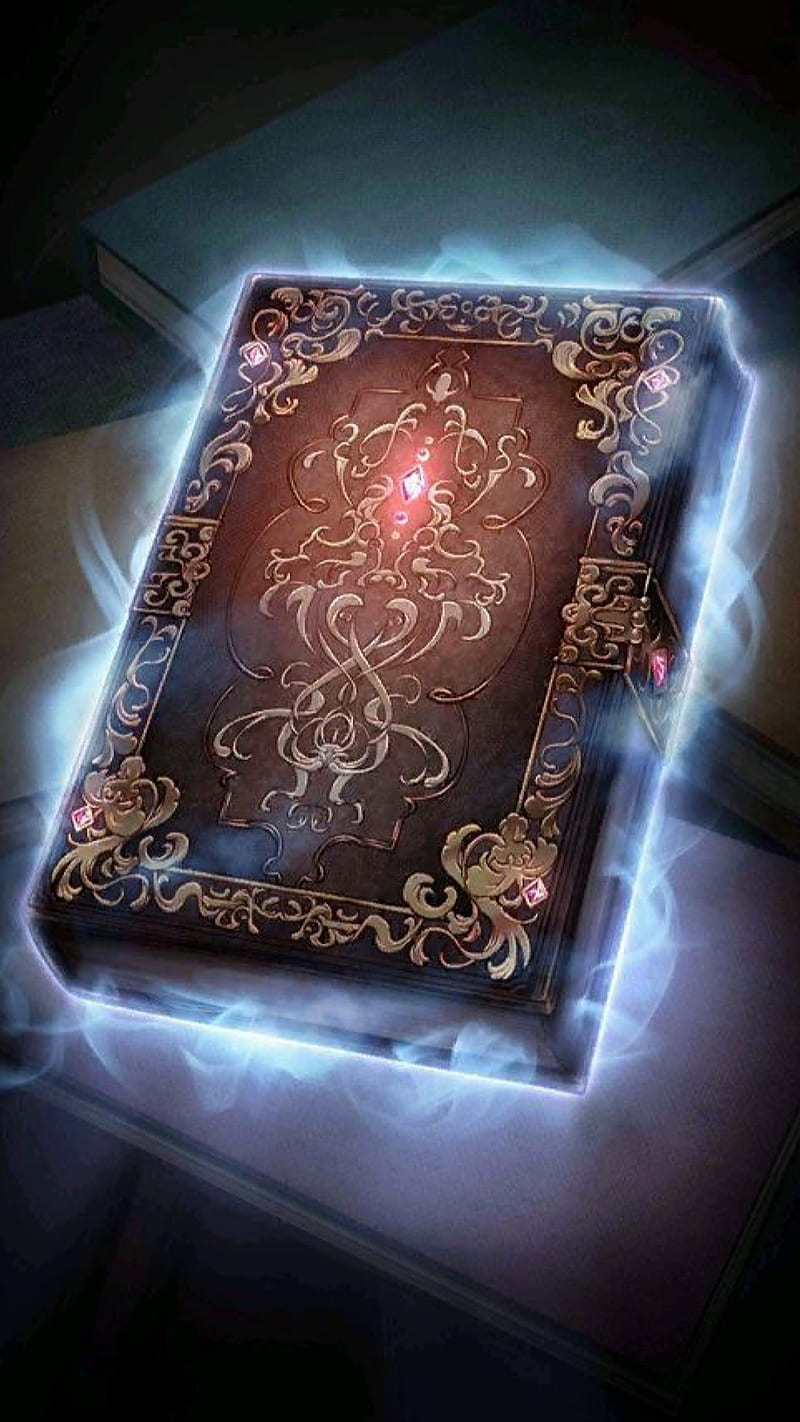Depicted in the illustration is an enchanting book, seemingly levitating above a stack of ordinary books. Bathed in an ethereal light, the book exudes a magical aura, further enhanced by its floating state. The cover, adorned with intricate engravings and glowing gemstones, features a significant lock on the right side, emphasizing its secrecy and need for a key to reveal its contents. This mysterious tome emanates a radiant light from the center, complemented by an ambient mist and bursts of electricity that add to its otherworldly appearance. The entire scene is illuminated from below, casting a spiritual fog that underscores the book's powerful and enigmatic nature. Suitable for a fantasy or science fiction narrative, this visual conveys an object of immense and mystical significance, known perhaps only to those versed in magic.